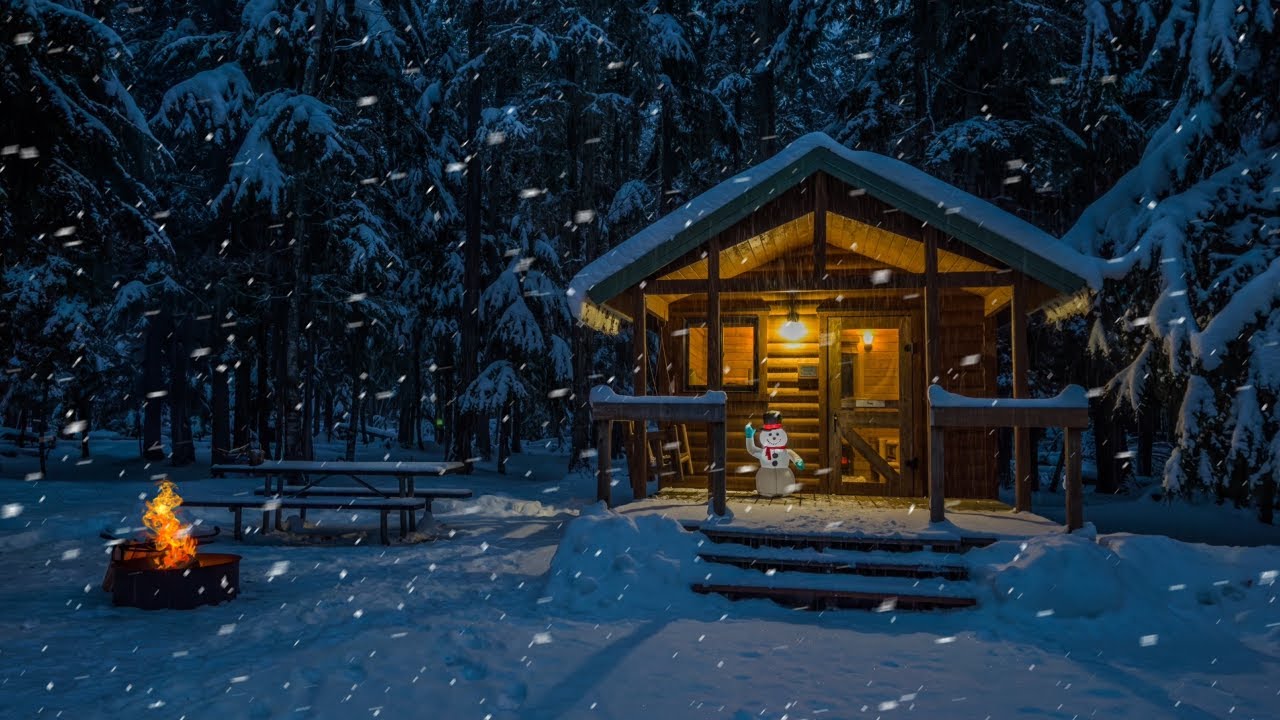The image depicts a cozy wooden cabin with a porch, nestled in a snow-covered landscape, adorned with evergreens that have snow on their boughs. It is nighttime, and snowflakes are gently drifting down, adding to the thick blanket of snow on the ground and the rooftop. The cabin is slightly to the right of center and features a glass front door, partially open, with a screen door as well. The warm glow from the porch light and interior lights shines invitingly, suggesting a welcoming and warm interior with cathedral ceilings. 

On the porch, a lit inflatable snowman stands cheerfully with one hand up, as if waving, dressed in a hat with a red rim, buttons, and a face. The porch, accessible via three steps, includes a single railing at arm height and a window to the left of the door. To the left of the cabin, there is a picnic table covered in snow and a campfire blazing in a fire pit. A bench sits near the fire, allowing for a cozy spot to enjoy the warmth amidst the snow. Surrounding the scene are numerous trees, completing this picturesque winter wonderland.